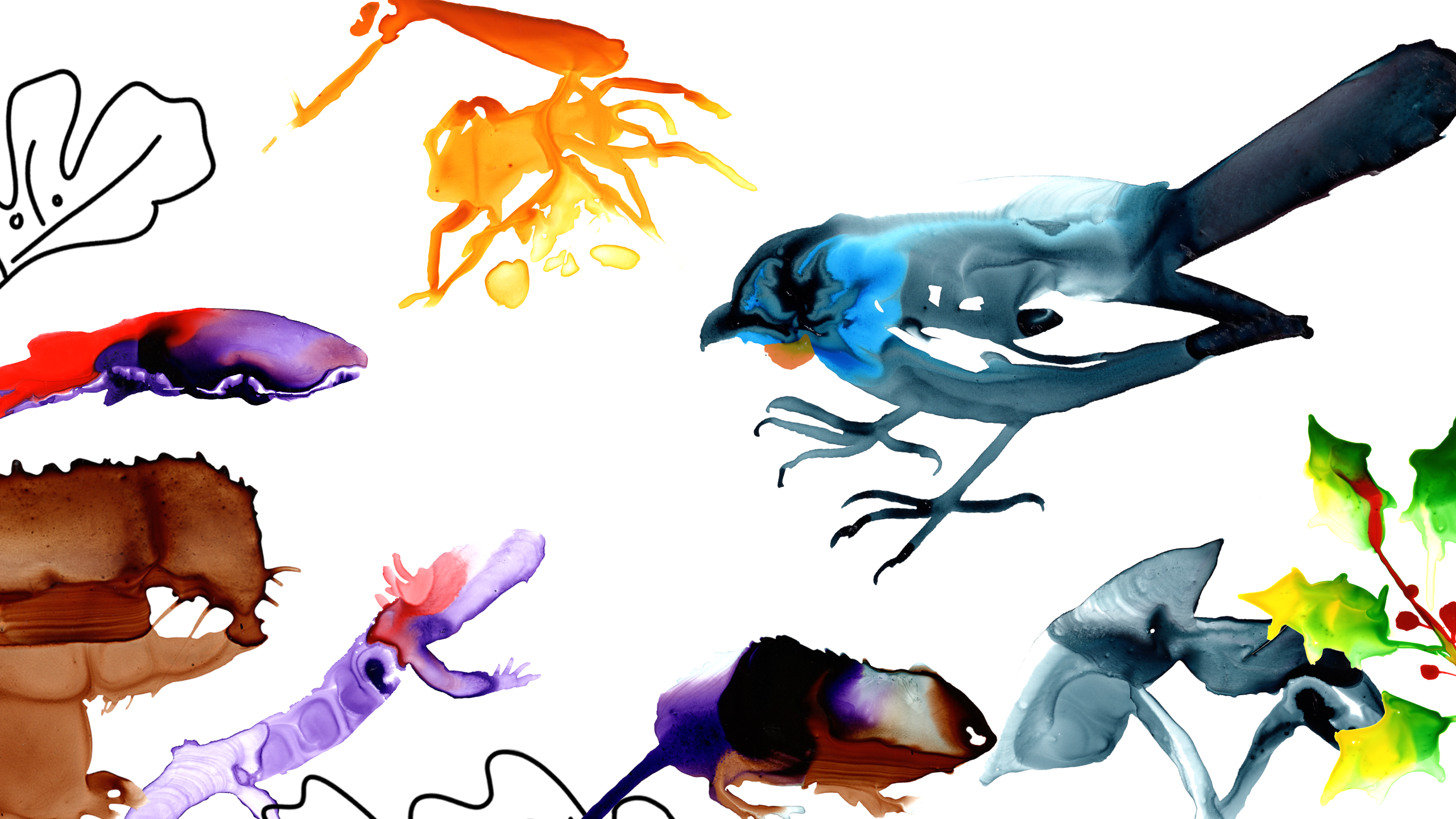The horizontally aligned, rectangular painting appears to be done with watercolors on a white background, depicting an abstract arrangement of various animals and elements. Dominating the center-right of the image is a bird, characterized by a black beak, with bright blue on its face, a blue upper body, and dark blue or black tail feathers. Below the bird, in the lower right corner, is a reptile-like creature that is green and interacts with a plant featuring bright green leaves and a brownish stem. Situated in the lower middle is a rodent, possibly a squirrel, with a blend of purple, black, and brown colors. To the lower left, there's a purple and red dragon-like figure, its mouth agape, sitting near a cliff drawn in brown. Rising above this area is a purplish-red fish. Additionally, an abstract, black-outlined leaf with a face is positioned in the top left corner, contributing to the whimsical and fantastical feel of the painting.